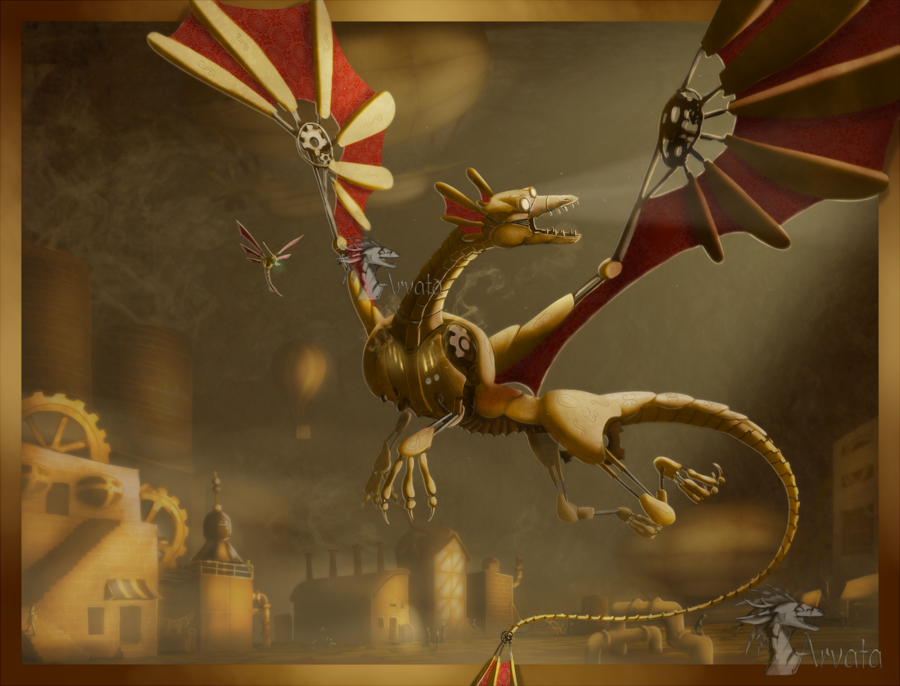The image depicts a computer-generated graphic of a mechanical dragon in flight, rendered in a detailed, industrial-fantasy style. The dragon, characterized by its metallic body and mechanical wings adorned with sprockets and chains, exudes an unmistakably robotic essence, further emphasized by visible gears and metal tendons within an open section of its abdomen. Its long, forked tail trails below as it flies, mouth agape to reveal sharp, menacing teeth. Predominantly hued in murky browns and golden shades, the environment enhances the dystopian atmosphere. In the background, other similar dragons can be seen flying against a nighttime sky tinged with gray and gold. The setting features factories with gears, smokestacks, and intricate piping, underscoring the industrial aesthetic. Buildings on the ground are sand-colored and dotted with large gears, reinforcing the futuristic, negative utopian scene. Additionally, the right corner of the image contains text, likely the artist’s signature, adding a personal touch to the illustration.